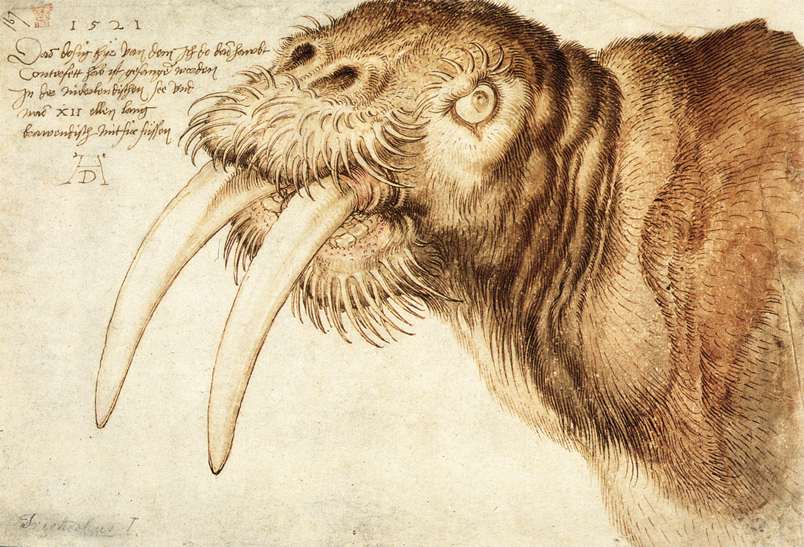The image features an intricately detailed drawing of a walrus with two large, downward-pointing tusks. The walrus has haunting white eyes and displays varying shades of brown fur, adding texture to its depicted form. Surrounding the walrus's mouth and chin, the fur is particularly dense and elongated, enhancing its imposing, almost psychotic expression. The background, resembling light gray or tan paper, hosts several additional elements: in the top left corner, "1521" is inscribed in brown, tightly-written cursive, accompanied by a paragraph in an unfamiliar language. The bottom lower left corner contains a faded, nearly illegible signature, while a logo that appears to merge an "H" and a "D" is situated at the bottom. Overall, the striking illustration of the walrus is rendered in black, brown, and light white ink, contributing to its eerie and captivating presence.